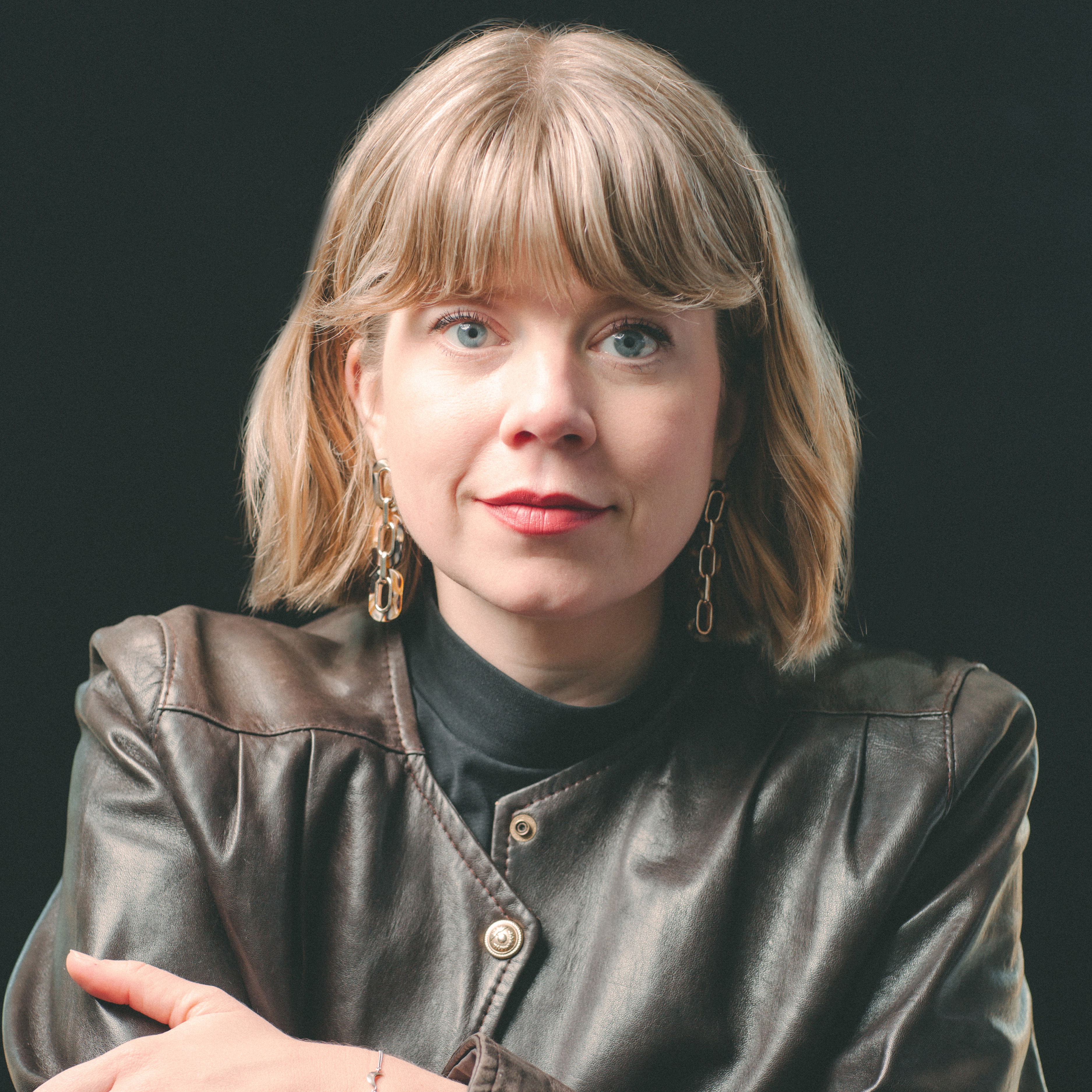This image showcases a striking portrait of a woman with shoulder-length, blonde hair and matching blonde bangs. Her eyes are a captivating bluish-gray, and she wears bold red lipstick, paired with a subtle, confident smirk on her lips. Adorning her ears are unique earrings, each designed with three small gold chain links. She is dressed in a chic brown leather jacket layered over a black shirt. The composition frames her from the chest up, with a deep black background that accentuates her features and outfit. A small glimpse of her hand is visible in the bottom left corner, suggesting her arms might be crossed, although only a portion of one arm can be seen.